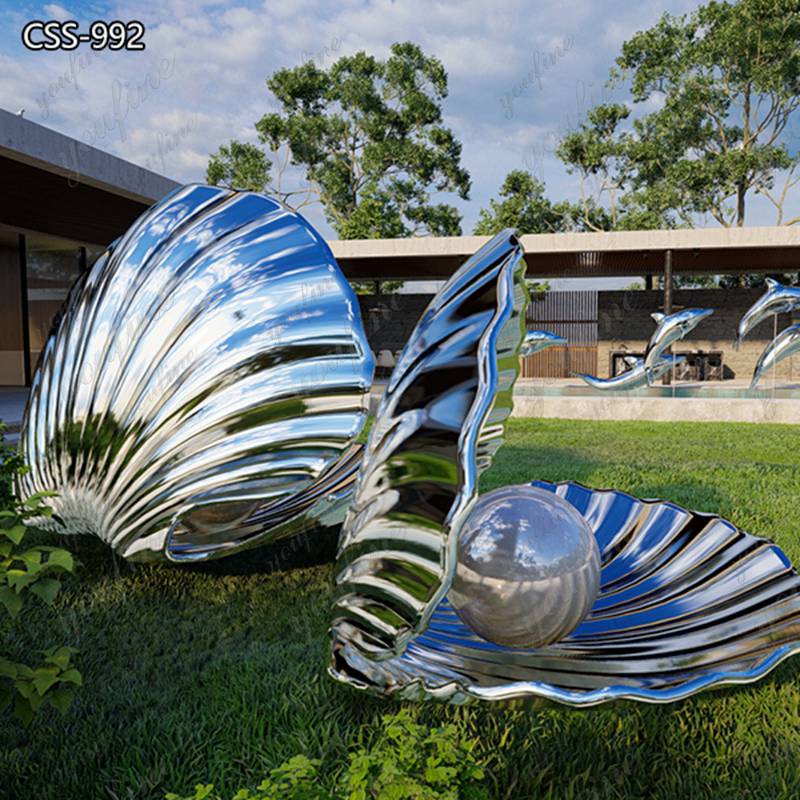This is an outdoor, square-colored photograph taken during the daytime, measuring approximately six inches by six inches. The bottom half of the image shows green grass interspersed with touches of green ivy. Sitting atop the grass are two large, silvery, reflective statues shaped like clamshells. The clamshell on the left is positioned slightly higher and further back, displaying its round scallop shape from the rear. The clamshell on the right, however, is open, revealing a large circular pearl within.

In the background, at the center of the photograph, stands an L-shaped, flat-roofed building featuring glass windows. To the right, there are statues of five silver dolphins, seemingly leaping through the air, likely supported by poles, implying a dynamic display, possibly a part of a pool area. The top of the photo showcases a cloudy blue sky with green trees visible in the upper left corner.

Overlaying the image, in the upper portion, is white text with a black outline reading "CSS-992." Across the photograph, there is a light gray cursive watermark, though its exact wording appears somewhat unclear and possibly reads "U-F-I-R-N-E." The polished metal statues and the modernist architectural elements suggest that this scene could be part of an Oceanic Museum or a similarly themed exhibition.